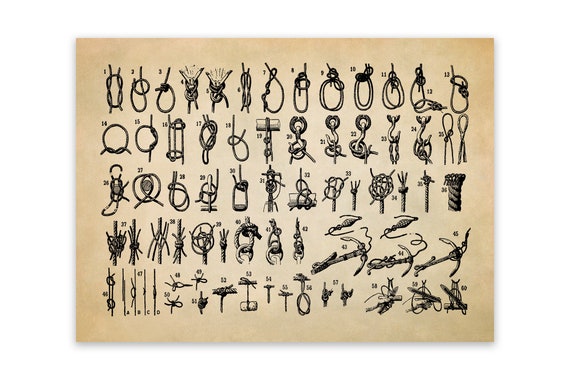This horizontally aligned, vintage chart on yellowed, beige parchment showcases 60 intricately hand-drawn nautical knots, meticulously arranged in five rows. Each row contains images numbered sequentially: the first row from 1 to 13, the second from 14 to 25, the third from 26 to 36, the fourth from 37 to 45, and the final fifth row from 46 to 60. The knots, varying from simple to highly complex formations, include those used for mooring boats, securing sailing vessels, knotting onto hooks or anchor chains, and preventing rope fraying. Alongside the knots, there are clear illustrations for stopping the fraying end of a rope and various anchoring techniques. In the lower section, there are also three diagrams demonstrating how certain knots can attach to a crossbow. The detailed and practical knots illustrated on this piece are just a small fraction of the over 6 billion unique knots identified by mathematicians.